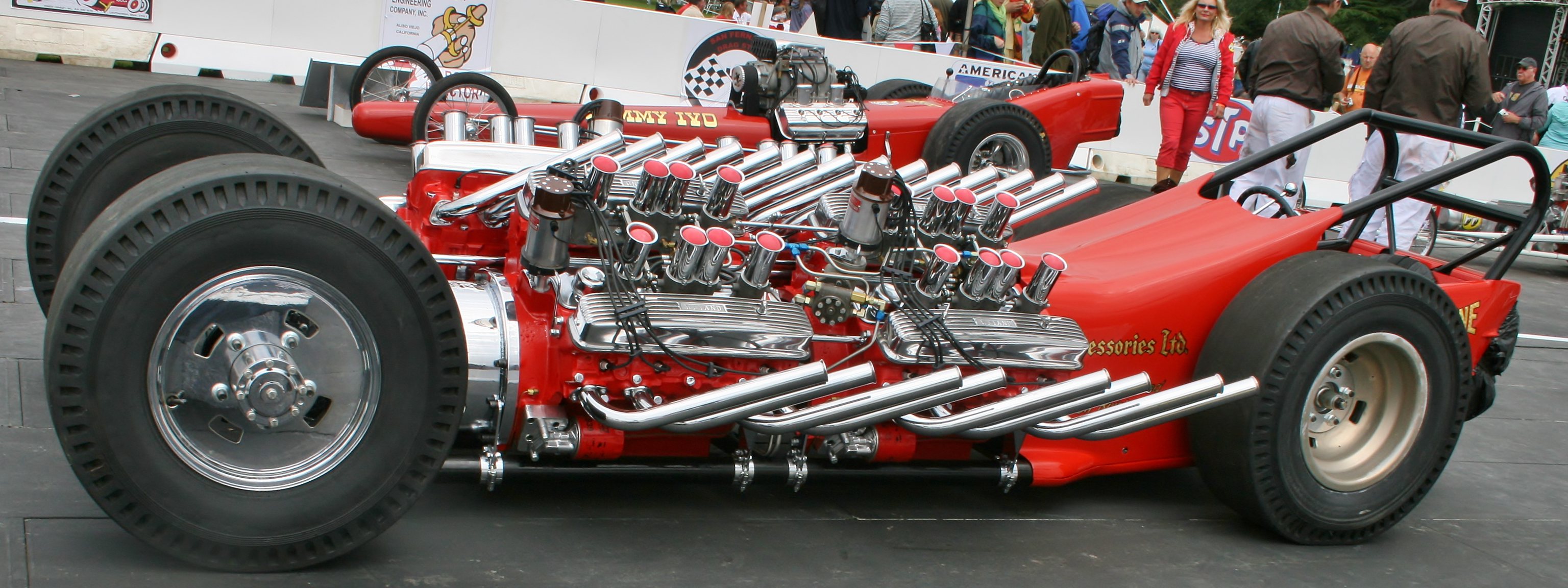This photograph captures a thrilling moment on a race track with two notable red drag racing cars, side-by-side. Both vehicles are heavily modified and adorned with large advertising stickers, emphasizing their competitive nature. The car on the left stands out with an exposed, elaborate engine featuring numerous silver pipes curving backwards, a testament to its high-performance design. This car has exceptionally large tires both at the front and rear, enhancing its stability and grip during high-speed sprints. The adjacent car, also red, contrasts with thinner front tires and a more streamlined appearance, but still boasts extensive mechanical modifications.

In the background, a wall separates the track from the enthusiastic spectators. Among them, a woman in a vivid red jacket and matching pants approaches the cars, accompanied by two men in brown jackets and white pants. The casual interaction of these individuals adds a human element to the scene, set against the mechanical marvels on display on the race track.